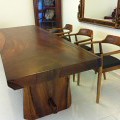In this intricate, very small photograph, roughly around an inch by an inch, you see part of a room that could be a boardroom or a classroom. Dominating the image is a substantial, heavy wooden table made from a single slab of darker wood. The table is beautifully crafted, exhibiting a rich wood grain with swirls of lighter colors. It is supported by thick slab legs, approximately three-quarters the width of the table itself. Positioned behind the table are three wooden chairs with a similar darker wood finish. These chairs feature flat lower backs, curved arms, and black leather upholstered cushions. The walls in the background are light-colored, possibly white or yellow, and the floor appears to be light or gray. On the wall behind the table, there is a large mirror with a gilt frame. In the back corner of the room, there is a tall curio cabinet or shelving unit containing various objects, possibly plates or items with blue accents. The room is sparsely furnished, drawing focus to the substantial table and chairs.